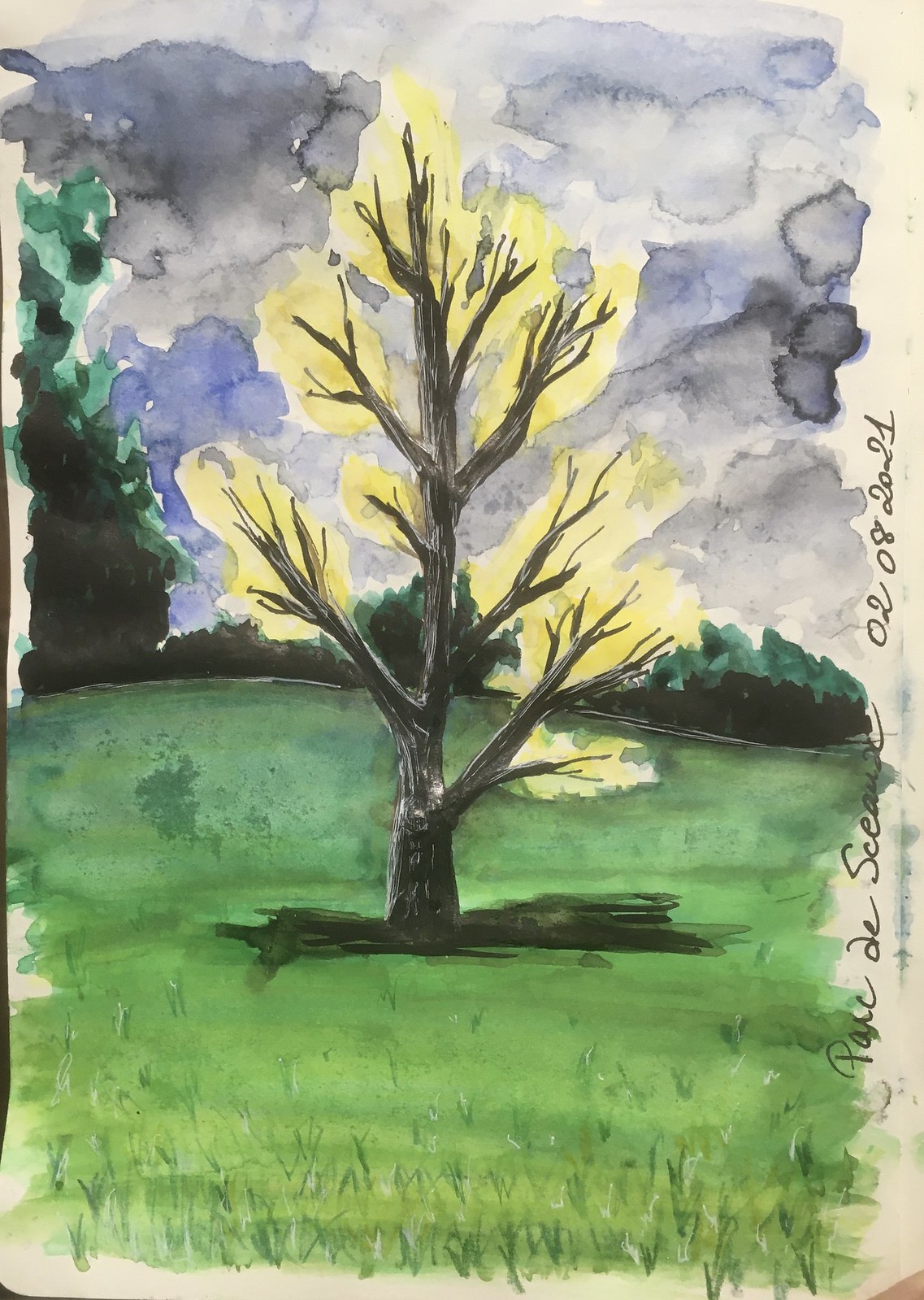A stunning watercolor painting from 2021 depicts a vibrant and serene natural scene. The ground is lush and green, with various hues of grass sprouting from it, adding depth and texture to the foreground. Dominating the center is a majestic tree with striking black wood; its branches extend gracefully in multiple directions – to the right, left, top right, and top left. At the ends of some branches, delicate yellow flowers bloom, providing a beautiful contrast against the dark branches. To the left of this central tree is another tree, this one verdantly green, accompanied by green bushes that add a rich layer of foliage to the composition. The background sky is a mesmerizing blend of light blue, dark blue, and white, creating a peaceful ambiance that envelops the entire scene.